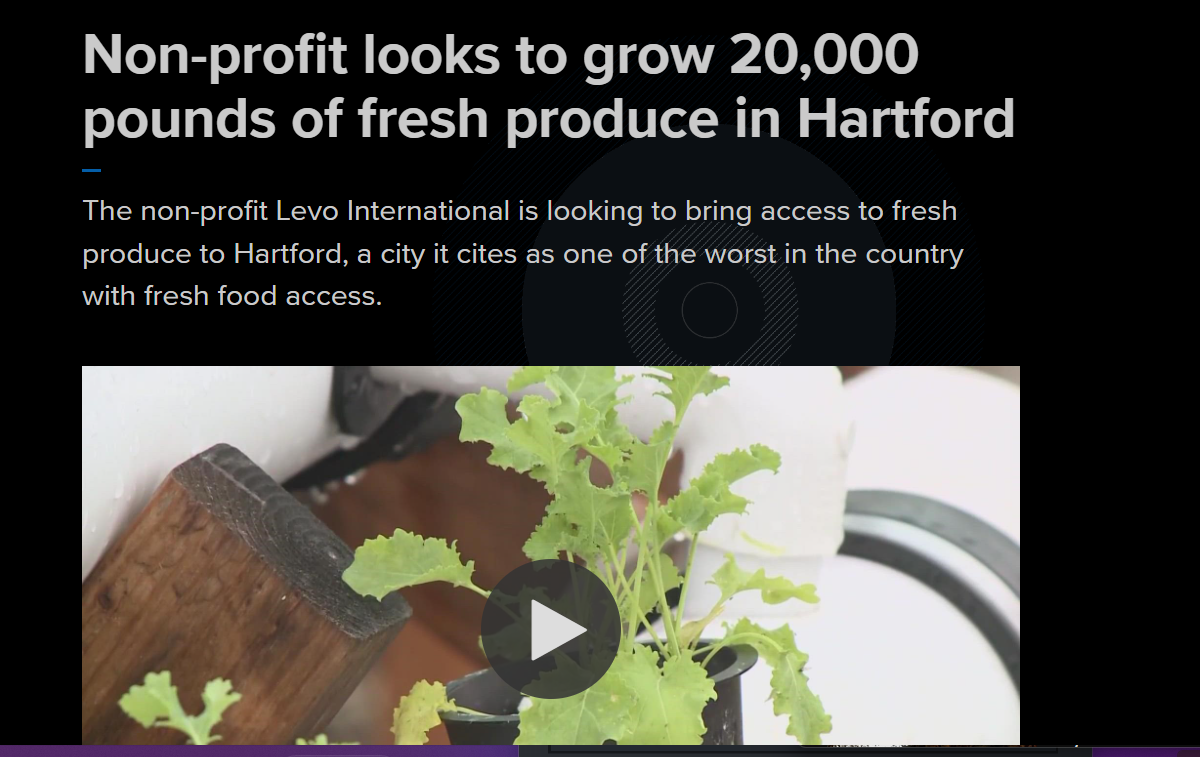This landscaped photo, resembling a news article, has a black background embellished with a patterned circle at the center. This circle initiates with a large, gray outer rim transitioning into a diagonal line pattern of white marks over gray, a smaller gray circle, and a white outline surrounding another gray ring. Dominating the top section of the photo, a bold white headline reads: "Non-profit looks to grow 20,000 pounds of fresh produce in Hartford." 

The article highlights Levo International's commendable initiative to enhance fresh produce access in Hartford, a city recognized for its limited fresh food availability. Centrally placed beneath the headline is a rectangular image portraying a green, leafy plant with thin, bright green stems. Despite a slight droop, the plant appears overall healthy. This image, adorned with a transparent play button featuring a white, right-facing triangular arrow, suggests that the visual is a video still. Adjacent to the plant, a dark brown plank rises, contrasting with some indistinct white objects in the blurred background.